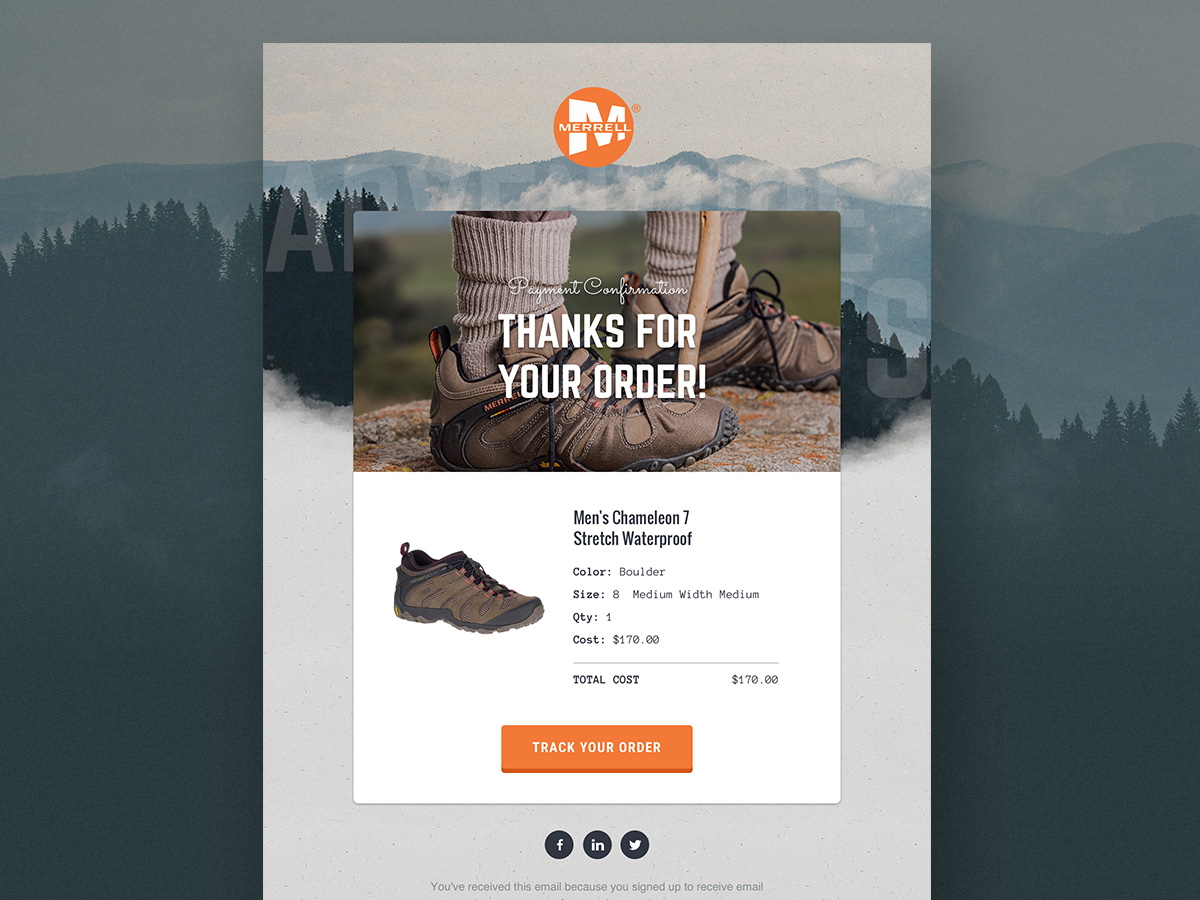The edited image features a desaturated background with a gray tint, showcasing a mountain range, a sky, and the silhouette of a forest on the mountainside. The central portion of the image contrasts with a pinkish-gray tint, appearing more transparent compared to the opaque border. Prominently displayed in the center is an orange circle with the letter "M" inside, accompanied by the word "Merrill."

Beneath this, there's a square image depicting a person's lower legs, from the ankles down, wearing gray tube socks and hiking shoes. Bold white capital letters next to this read, "Thanks for your order." Below this section is a stock photo of one of the hiking shoes with the following description: "Men's Camellia 7 Stretch Waterproof, Color: Boulder, Size: Small/Medium, Width: Medium." To complete the image, there is an orange "Track Your Order" button at the bottom.